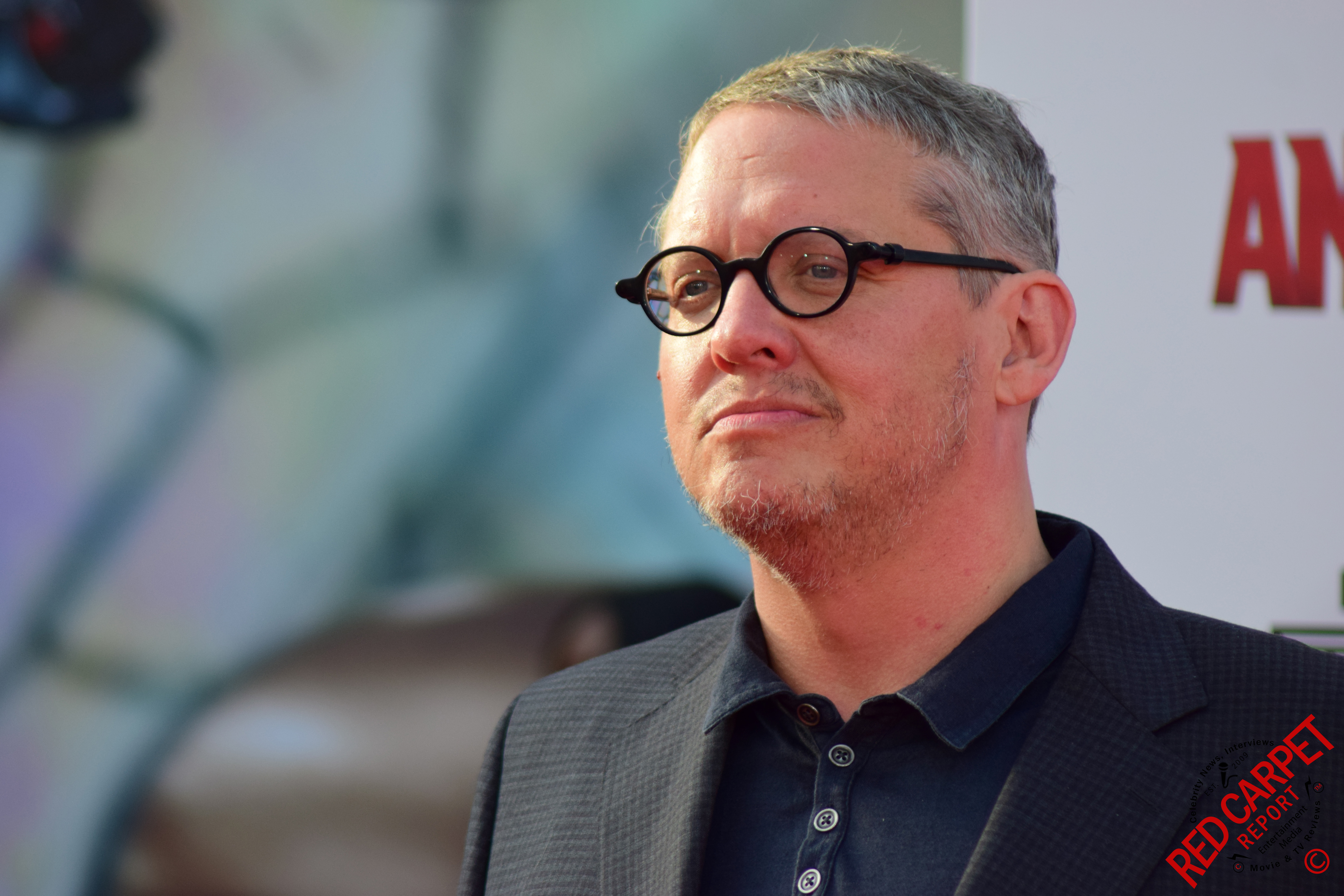This detailed photograph captures a middle-aged white man with fair skin, short gray hair, and blue eyes. He is wearing black round eyeglasses and has a neatly trimmed, slightly messy facial hair. The man is dressed in a navy blue polo shirt paired with a black suit jacket. He is positioned slightly to the right of the image, with the shot capturing him from the chest up at a slight angle from his left side. His expression features a subtle smirk, with his lips slightly curving to one side.

Behind him, towards his left shoulder, there is a white background featuring text and some faint colors, including blue and red, implying the presence of a poster or a back wall. The red text prominently reads "Red Carpet Report". The rest of the background, especially over his right shoulder, appears blurred and indistinct, with hints of white, red, and brown colors, potentially suggesting a lively environment, possibly an event like a movie premiere. Light from the outdoor setting casts a bright shine on the right side of his forehead and face, enhancing the overall high-energy ambiance of the photograph.